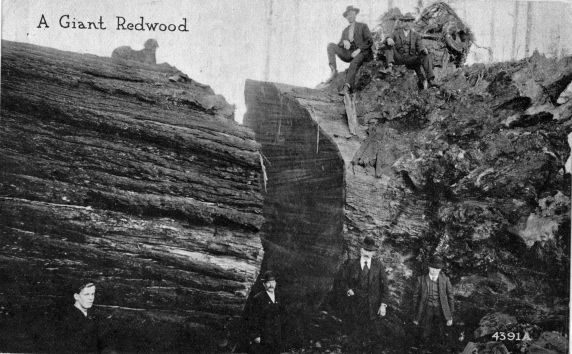This horizontally aligned rectangular black and white photograph features a prominent, horizontally positioned giant redwood tree trunk that consumes much of the image. The upper left-hand corner displays the text "a giant redwood" in dark gray print, while the lower right-hand corner is marked with the identifier "4391A" in gray. The scene is set against a light gray background suggestive of a heavily forested area, discernible by the vertical lines indicative of smaller tree trunks.

Perched atop this colossal log is a man dressed in a suit and hat, exhibiting the era's fashion. Notably, there is also a dog on the fallen tree, adding a touch of companionship to the scene. Below, on the ground adjacent to the log, stand four more men, all similarly attired in suits, ties, and hats, further underscoring the period setting of the photograph. The overall atmosphere, with its grayscale hues and attire, evokes a sense of a bygone era, possibly several decades ago, accentuating the historical significance of the image.